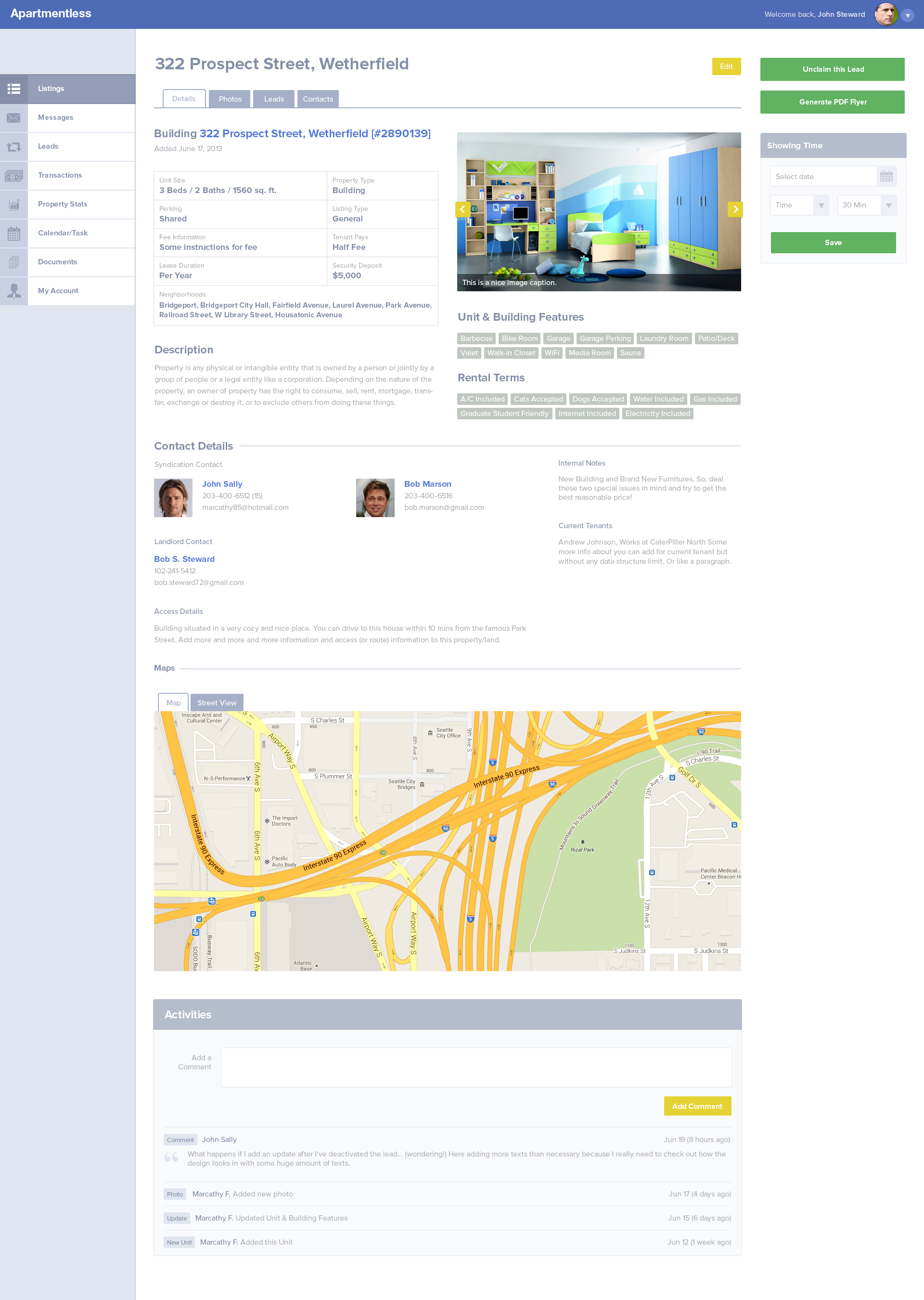**Detailed Property Listing Overview for 322 Prospect Street, Weatherfield**

**Program Source: Apartment Lists (Apartmentless)**
**User: John Stewart**

---

**Property Details:**
- **Location:** 322 Prospect Street, Weatherfield (W-E-T-H-E-R-F-I-E-L-D), ZIP: 2890139
- **Type:** Building
- **Unit Size:** 3 bedrooms, 2 bathrooms, 1560 square feet
- **Parking:** Shared
- **Rental Terms:**
  - **Security Deposit:** $5,000
  - **Lease Duration:** Per year
  - **Fee:** Tenants pay half of the fee
  - **Listing Type:** General

**Property Description:**
This property at 322 Prospect Street in Weatherfield features a spacious unit with three bedrooms and two bathrooms, totaling 1560 square feet. The building offers shared parking facilities. 

The neighborhood encompasses notable areas such as Bridgeport, Bridgeport City Hall, Fairfield Avenue, Laurel Avenue, Park Avenue, Railroad Street, W Library Street, and House Tonic Avenue. This makes the location convenient for both residential and commuting purposes.

**Additional Information:**
- **Unit Features:** 
  - Recently built structure
  - Brand new furnishings

Potential tenants should note the specific conditions related to this new development and aim for competitive pricing. The current tenant, Andrew Johnson, is employed at Caleb Pilter North.

**Contact Information:**
- **Syndication Contacts:**
  - John Sally: 203-400-6512
  - Bob Mason: 203-400-6516
- **Landlord Contact:**
  - Bob S. Stewart: 102-241-5412 
  - Email: bob.steward72@gmail.com

For more precise location details, a map is included to visualize the property in its immediate surroundings.

---

**Available Links (Displayed to the Left of the Listing):**
- Listing Link
- Messages
- Leads
- Transactions
- Property Stats
- Calendar Tasks
- Documents
- Mile Count Option

**Property Usage Rights:**
Owners have the rights to consume, sell, rent, mortgage, transfer, exchange, or destroy the property, or exclude others from these actions based on ownership rights.

This detailed description aims to provide comprehensive information regarding the property at 322 Prospect Street, ensuring potential tenants have all necessary details to make an informed decision.